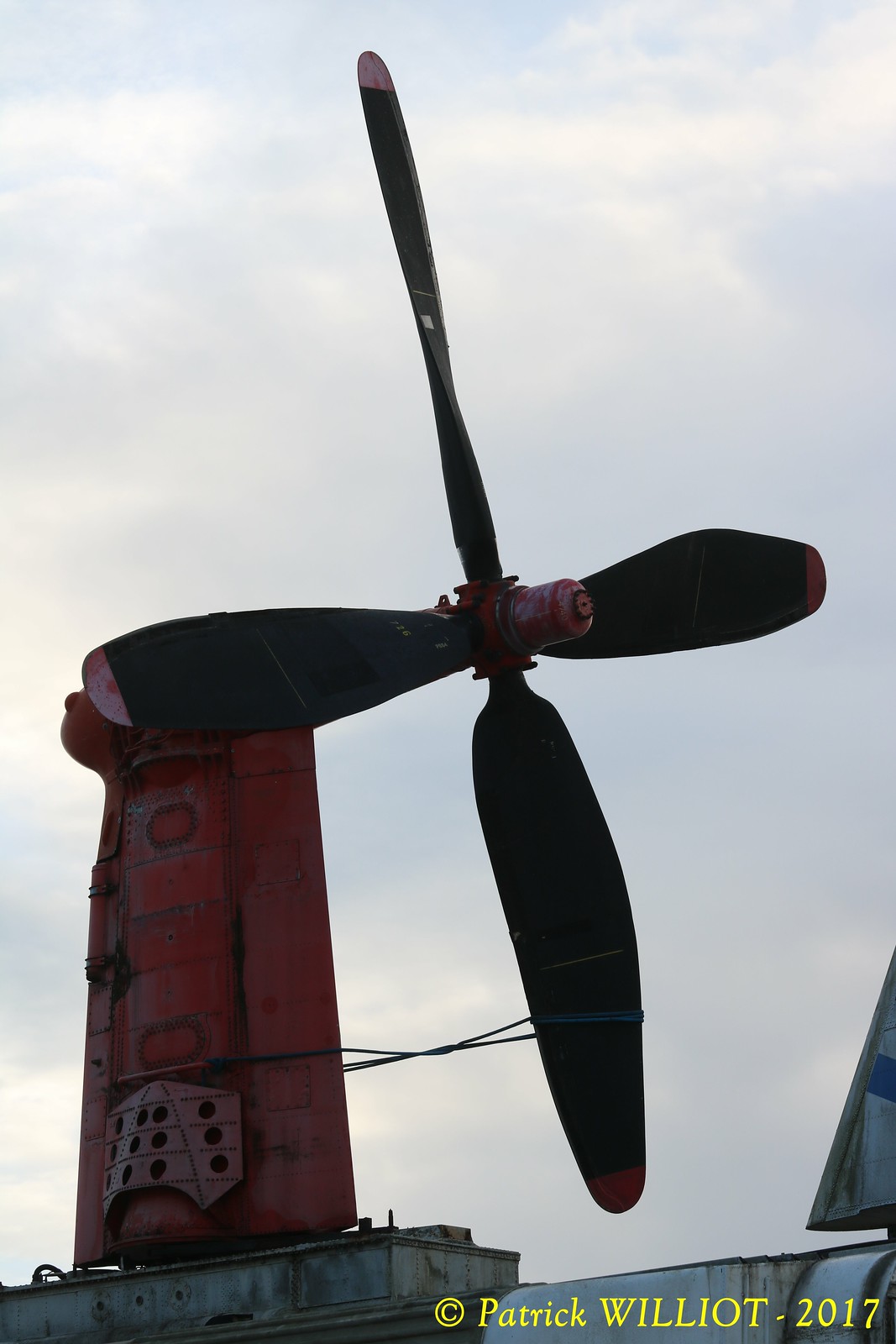The image features a close-up of a small, four-bladed windmill or turbine. The black blades are distinctively tipped in red. At the center of the turbine is a cylindrical red piece, attached to a larger cylindrical structure that tapers down into an almost square-like shape, with rounded top and bottom edges. The red cylinder on the left side bears a pink figure with black dots, resembling a partially cut-off D20 die, showing 12 black dots separated by small dotted black lines. The turbine is mounted on a gray structure, possibly a craft of some kind, which is not fully visible. The background consists of a grayish blue sky dotted with white clouds. At the lower right corner of the image, the text “© Patrick Williot - 2017” is written in small yellow letters.